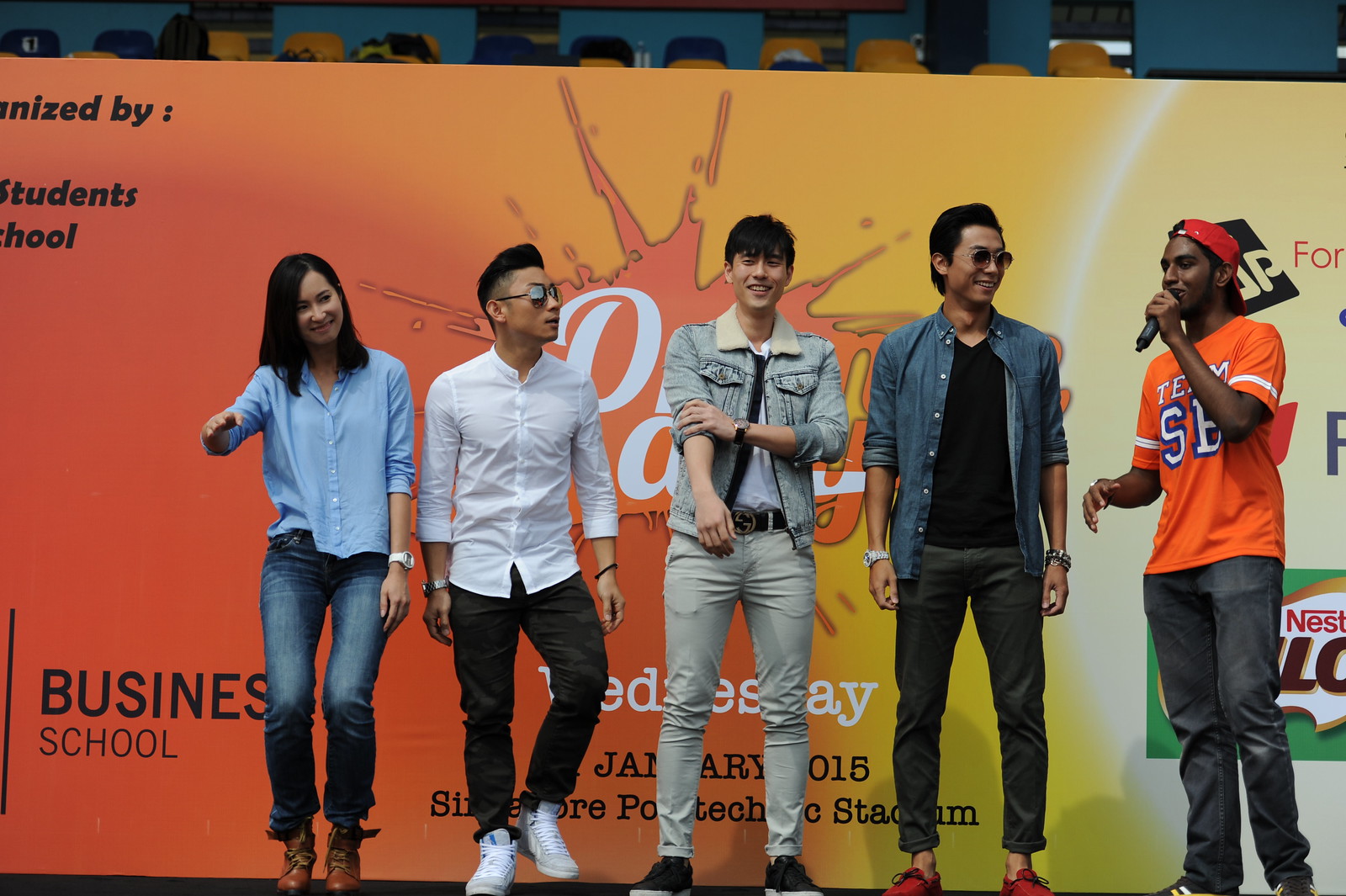The image depicts five young Asian individuals on a stage, likely students from Singapore Polytechnic, as indicated by the partially visible backdrop text. The colorful backdrop features a large sign with red, yellow, and green hues that says "Business School," "Wednesday," "January 2015," and possibly "Singapore Polytechnic Stadium," though some words are obscured by the figures. The woman on the far left, wearing blue jeans and a long-sleeve blue button-down shirt with a white watch, has shoulder-length straight black hair, and is extending her right arm forward, seemingly dancing. To her right is a man with shaved sides and taller, combed-back black hair, wearing sunglasses, a white button-down shirt, black pants, and white tennis shoes. The middle man, smiling at the camera, sports light-colored blue jeans and a blue jean jacket, with short black hair and longer bangs in the front. Next to him is another man in a denim button-down shirt over a black v-neck shirt, dark gray pants, and red tennis shoes, smiling at the person beside him. The man on the far right, who appears to be giving a speech, is wearing a red baseball cap backwards, an orange and white team jersey, and dark gray pants while holding a microphone. The group appears cheerful and energized, engaging in movements and interactions that suggest they are enjoying themselves.